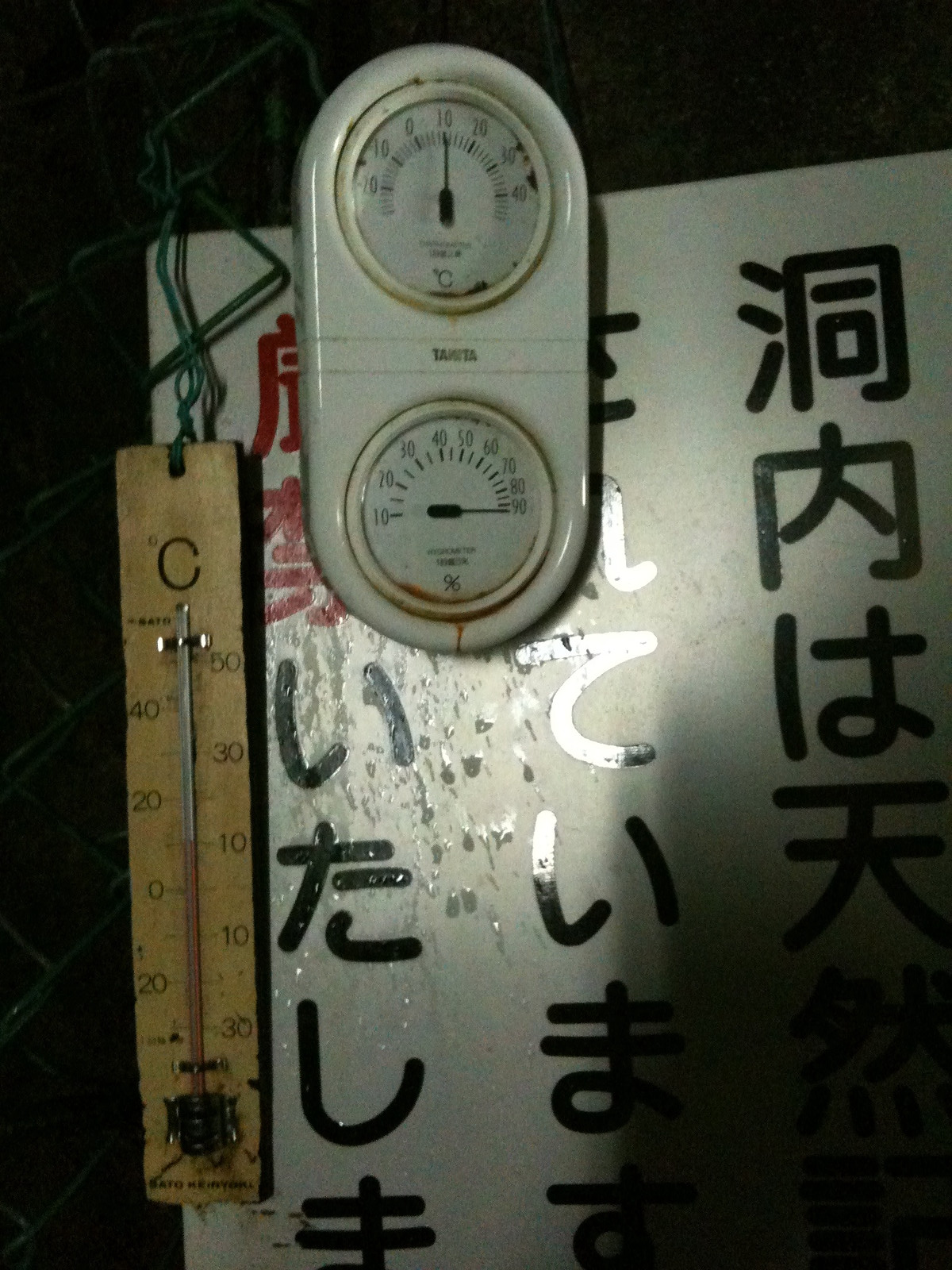The image features a complex assembly of elements, centered around a sign displaying a mixture of Asian characters—possibly Chinese, Japanese, or Korean—against a gray background with red and black text. Dominating the foreground is a long yellow thermometer, marked with a temperature scale ranging from -30 to 50 degrees Celsius, currently indicating approximately 10 degrees Celsius. This thermometer appears quite aged, with visible dirt and rust, and is attached with green string, casting a distinct black shadow behind it.

Adjacent to the thermometer is a circular white device, partially covering the sign. This device also features a temperature display, reinforcing the 10 degrees Celsius reading, and includes a lower section that measures humidity, indicated as a percentage. The face of the device has black text on a white background, with noticeable rust around its edges.

Overall, the image conveys a sense of wear and utilitarian function, set against a backdrop of Asian text and dark contrasting colors. The scene is visually anchored by the dual thermometers and their clear emphasis on temperature and humidity readings.